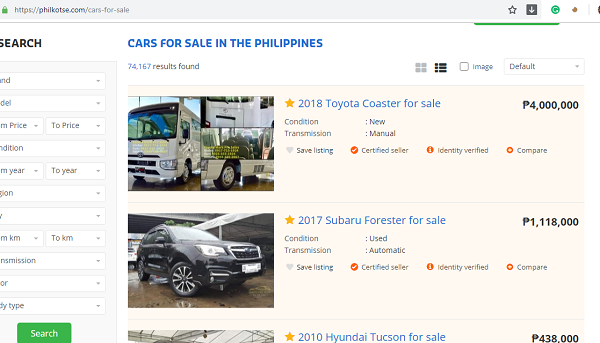This is a screenshot of the car listing website Philkotse.com, a popular platform for buying and selling cars in the Philippines. The website's logo and name are prominently displayed in the upper left corner of the page. On the left sidebar, the site offers an extensive filter system for refining car searches, featuring 11 dropdown menus. Users can specify criteria such as year, make, model, price range, condition, mileage, and transmission type. Below the filters, there's a green search button designed to initiate the query based on the selected parameters. 

In this instance, the user's specified criteria have generated 74,167 search results for cars available across the Philippines. The top listing is a 2018 Toyota Coaster, which appears to be a large motorhome, with an accompanying photo to the left of the listing. The asking price for this vehicle is ₱400,000. The second result is a 2017 Subaru Forester, also illustrated with a photo to its left, priced at ₱1,118,000.